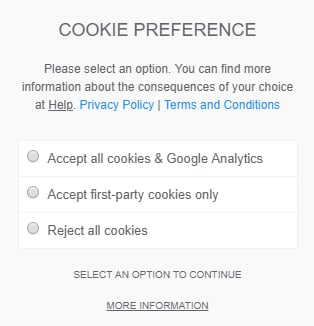The image displays a cookie preference pop-up, typically encountered when visiting a website. The pop-up features a gray background with traditional black text. At the top, "Cookie Preferences" is prominently displayed in a bold font. Below this, the text "Please select an option" is visible, followed by instructions for further information: "You can find more information about the consequences of your choice at help, Privacy Policy, and Terms and Conditions." The "Privacy Policy" and "Terms and Conditions" are highlighted in blue, indicating clickable links.

The pop-up offers three options for cookie preferences, each accompanied by a radio button. The choices are: "Accept all cookies and Google Analytics," "Accept first-party cookies only," and "Reject all cookies." None of the options are pre-selected. Additionally, there is a message stating, "Select an option to continue," emphasizing the necessity of making a choice to proceed. "More information" is underlined, suggesting that it is also a clickable link.

The pop-up appears to have been captured, possibly via a screenshot, and displays a plain, slightly grayed-out background behind the text elements. No specific website details are discernible from the image. The text "help" is also underlined, indicating another link, and the mention of Google Analytics includes a small, distinct symbol adjacent to it.